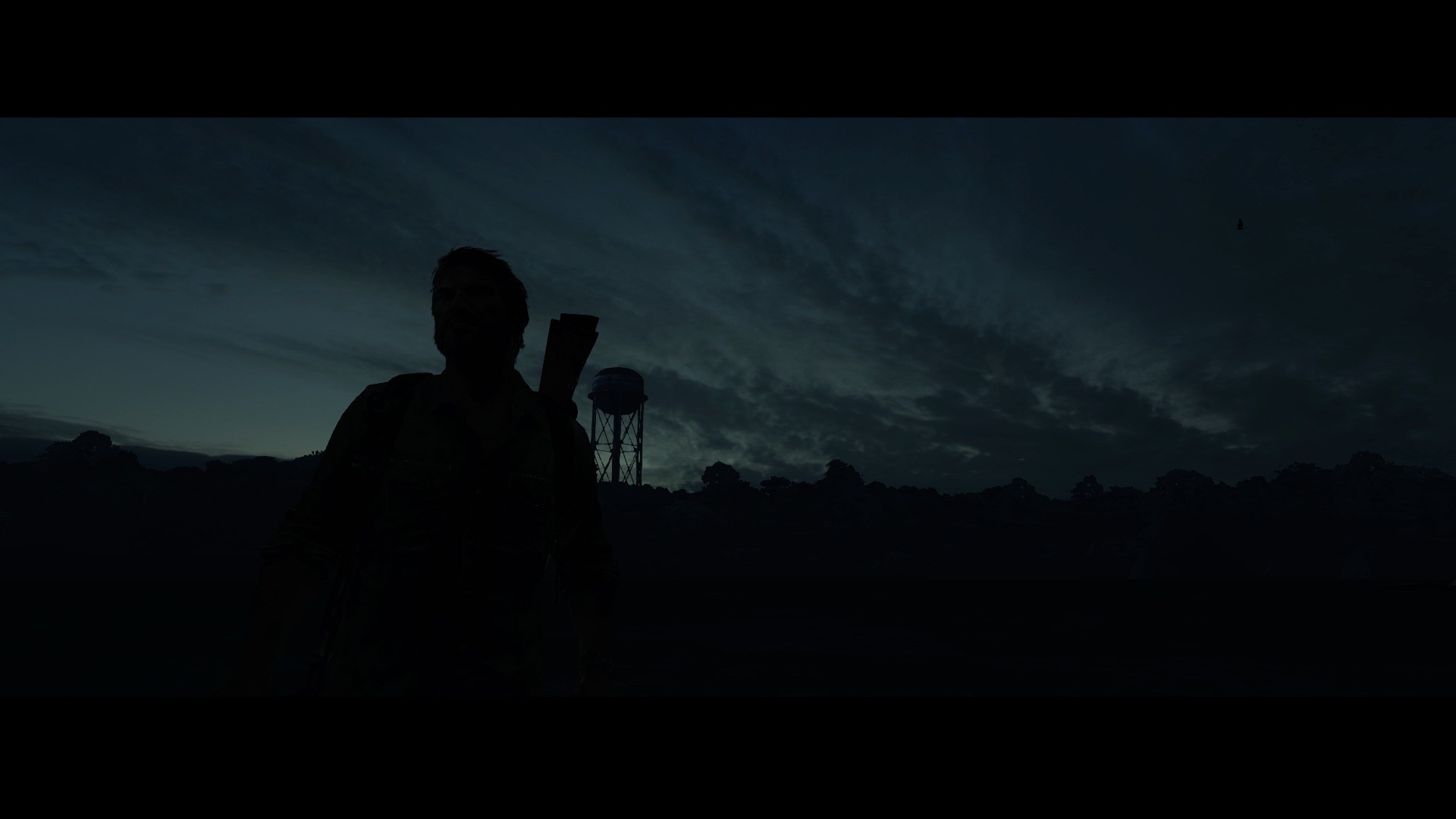The photograph is a striking, panoramic image with a width about twice its height, framed by pronounced letterboxing that takes up roughly 15% of the top and bottom of the picture. The scene is shrouded in very dim lighting, creating a predominantly silhouetted composition. The sky suggests a time just after sunset or right before sunrise, radiating a faint light over sparse hills and trees. It is a partly cloudy sky, with varying shades of dark grey clouds and a few clear patches. The left side of the image features the silhouette of a person, identifiable by their head and shoulders, positioned about a third into the frame. Approximately 10% left of center, a tall, slender water tower with its distinctive oval top and supporting legs rises against the dusky backdrop. Though the horizon line and tree silhouettes are barely discernible, they add a layer of depth to this night-time landscape.